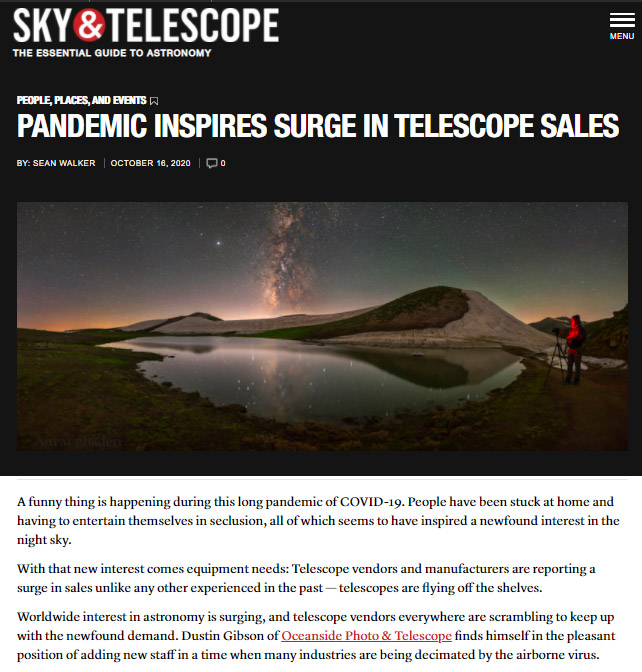The image features a predominantly black rectangle that gradually becomes lighter towards the bottom. Prominently displayed in white text at the top, it reads "Sky," followed by a red circle containing a white ampersand. The word "Telescope" is also in white. Below this, the subtitle "The Essential Guide to Astronomy" is written.

On the right side, three horizontal lines symbolize a menu button labeled "Menu," while the left side lists sections named "People, Places, and Events." Below this section, it reads "Pandemic Inspires Surge in Telescope Sales," credited to Sean Walker with a small white line underneath that states the date "October 16, 2020." Adjacent to this date is an icon resembling a speech bubble with a zero next to it, indicating no comments.

The main image depicts a picturesque scene of hills and a bit of water under a sky, showcasing an individual dressed in red standing beside a setup that likely includes a telescope. The caption beneath the image reads: 

"A funny thing happened during this long pandemic of COVID-19. People have been stuck at home and having to entertain themselves in seclusion, all of which seems to have inspired a newfound interest in the night sky. With that new interest comes equipment needs. Telescope vendors and manufacturers are reporting a surge in sales unlike any other experience in the past. Telescopes are flying off the shelves. Worldwide interest in astronomy is surging, and telescope vendors everywhere are scrambling to keep up with the newfound demand. Dustin Gibson of Oceanside Photo and Telescope finds himself in the pleasant position of adding new staff in a time when many industries are being decimated by the airborne virus." 

The name "Oceanside Photo and Telescope" is notably highlighted in red and underlined.